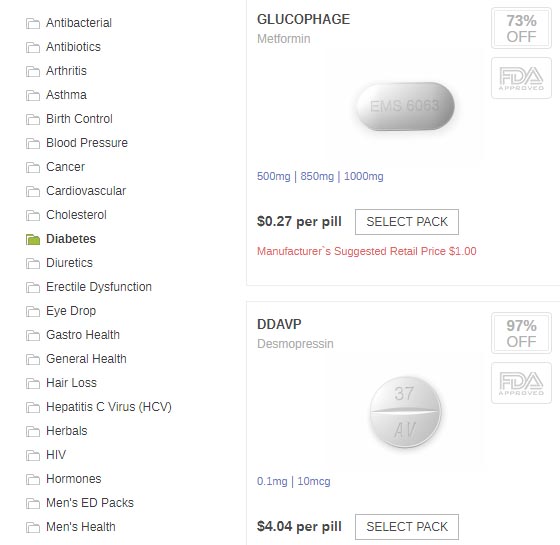The page provides information about various medicines classified by medical conditions, listed in the left-hand column. Types of conditions include antibacterial, antibiotics, arthritis, asthma, birth control, blood pressure, cancer, cardiovascular, cholesterol, with a highlighted focus on diabetes. 

In the right-hand column, the page details drugs specifically for diabetes. The first drug listed is Glucophage (metformin), accompanied by an image of a pill with EMS-6063 stamped on it. It offers three different potential dosages priced at 27 cents per pill, with a manufacturer-suggested retail price of $1 highlighted in red.

Beneath Glucophage, the drug DD-AVP (desmopressin) is displayed with an image of a circular pill stamped with 37-AV. It is priced at $4.00 or four cents per pill, with an option to select a pack.

The page emphasizes that these drugs are 97% off and FDA approved. The right-hand column also lists drugs and supplements related to other health conditions such as diuretics, erectile dysfunction, eye care, gastrointestinal health, general health, hair loss, hepatitis C, herbal treatments, HIV, hormones, men's ED packs, and men's health. Images of the respective drugs are situated on the right side of the page.